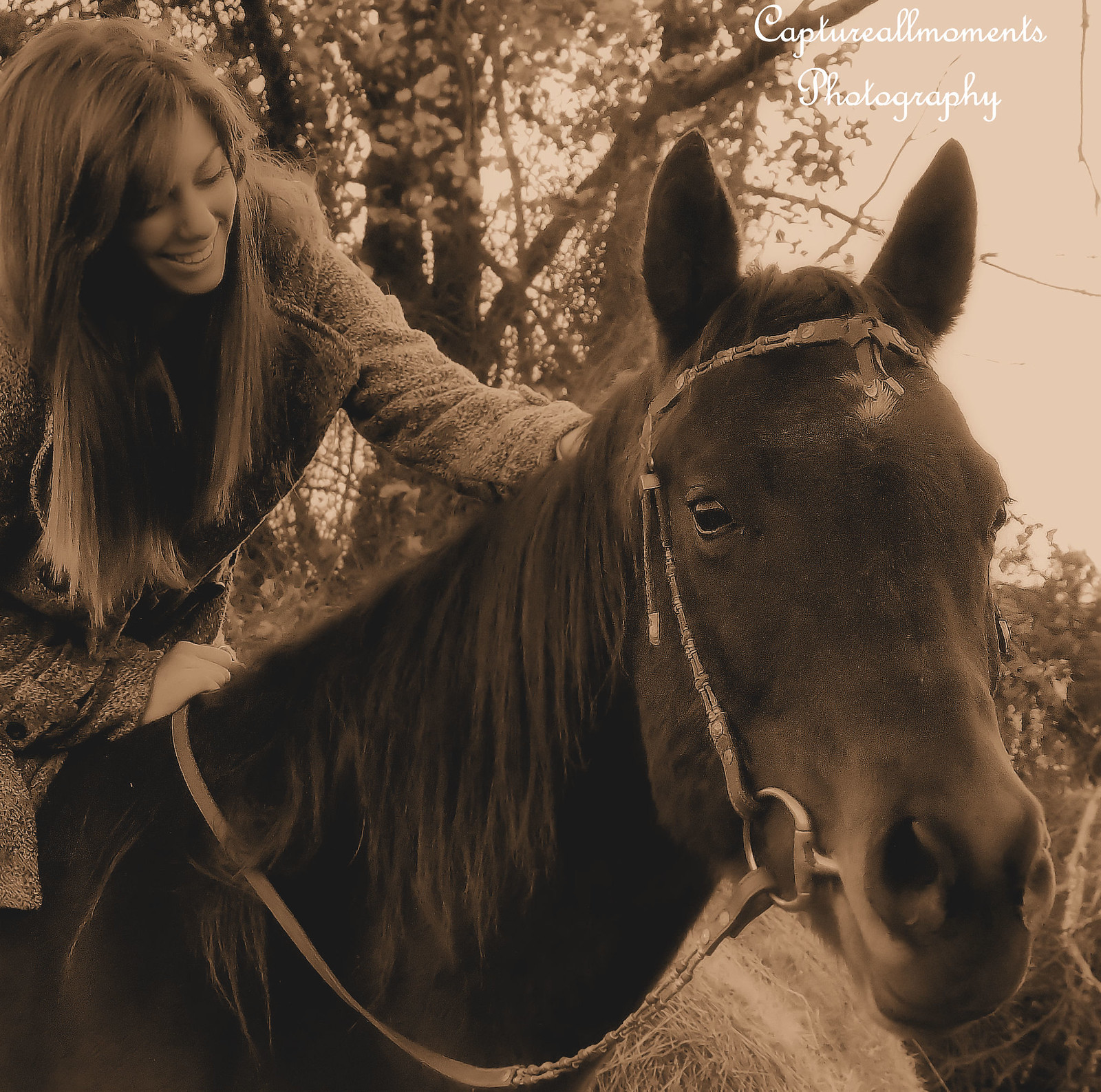In this sepia-toned photograph, a young blonde woman with long hair sits atop a dark-colored horse, smiling warmly as she leans over to pet its well-groomed mane. The horse is adorned with a bridle featuring reins and a bit, and it faces the viewer with its ears raised attentively. Both appear to be on a trail, suggested by the background, which includes trees and a bale of hay. The woman is dressed in a somewhat fancy coat, likely chosen for the photo shoot. The overall scene gives a vintage feel, enhanced by the brown and white monotone palette of the image. In the top right corner, white cursive text reads "Capture All Moments Photography," identifying the author of the photo.